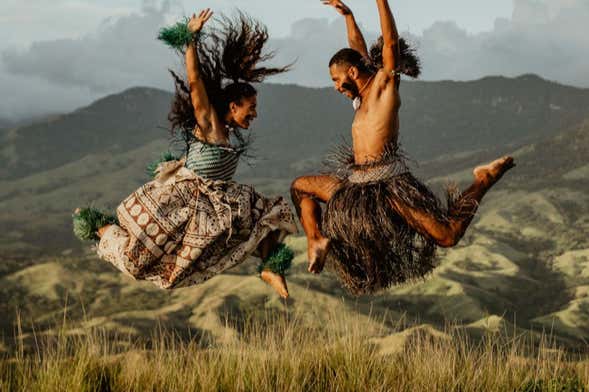The photograph captures a dynamic moment of two individuals dressed in traditional Polynesian-Hawaiian attire, jumping towards each other against a backdrop of rolling green hills and cloudy skies. On the right side of the image, the man is leaping into the air with his arms raised above his head, both feet completely off the ground. He wears a brown grass skirt, is barefoot, and has a large white shell necklace that dangles around his neck. His face is adorned with black paint, and his long dark hair flows behind him in a ponytail. His olive complexion, possibly enhanced by a tan, contrasts with the lighter color of his bare feet. 

On the left, the woman mirrors his leap, also barefoot, with her arms reaching upwards. She is dressed in a long white skirt with a brown print resembling a large tablecloth and a diagonally-striped blue and white shirt. Green fuzzy leis adorn her wrists and ankles, accentuating her vibrant movements. Her dark hair, smoothed back into a ponytail, flies up dramatically as she jumps. The scene is set on a grassy plain with patches of white sand dunes and mixed vegetation, against a backdrop of green mountains under a sky filled with white and gray clouds, giving the impression of an impending yet non-threatening storm. The vividness of their attire and the energy of their poses create a striking contrast with the natural landscape, suggesting a celebratory or ritualistic dance.